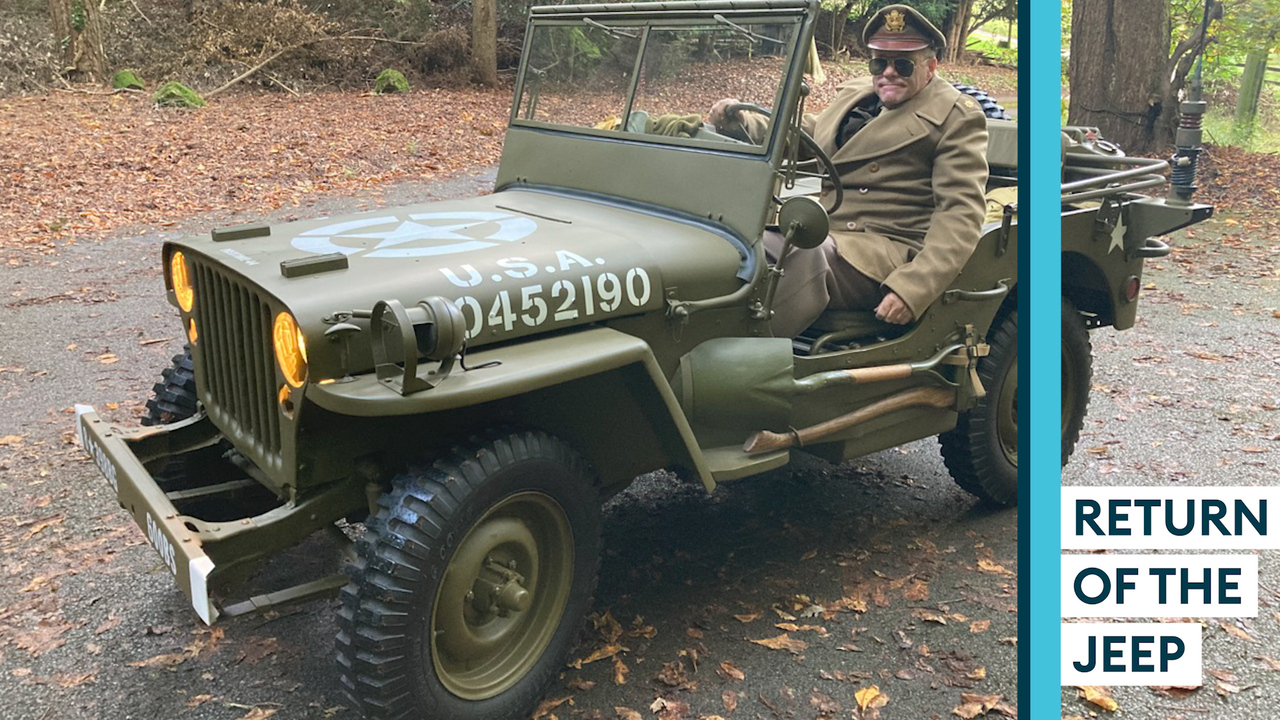In this detailed photograph, taken outdoors during daytime, a dark green military jeep is prominently featured on a road scattered with dry leaves. The jeep, which has distinct yellow headlights and a white star on its hood, bears the inscription "USA 0452190". A middle-aged man, dressed in a brown coat, pants, and an army cap—resembling a general or high-ranking officer—sits in the driver’s seat. With his right hand on the steering wheel and his left hand resting at his side, he gazes directly at the camera. Behind him, a shovel and a hammer are visibly attached to the jeep's side. The road is bordered by plants and more dry leaves, with trees in the background. Notably, the jeep appears stationary, oriented towards the left in a side-profile shot. The bottom right corner of the image features the text "RETURN OF THE JEEP," accompanied by a vertical line of alternating light and dark blue hues. The scene is rich with earthy and military tones, including shades of army green, yellow, tan, brown, and hints of red, set against the natural backdrop of the woodland surroundings.